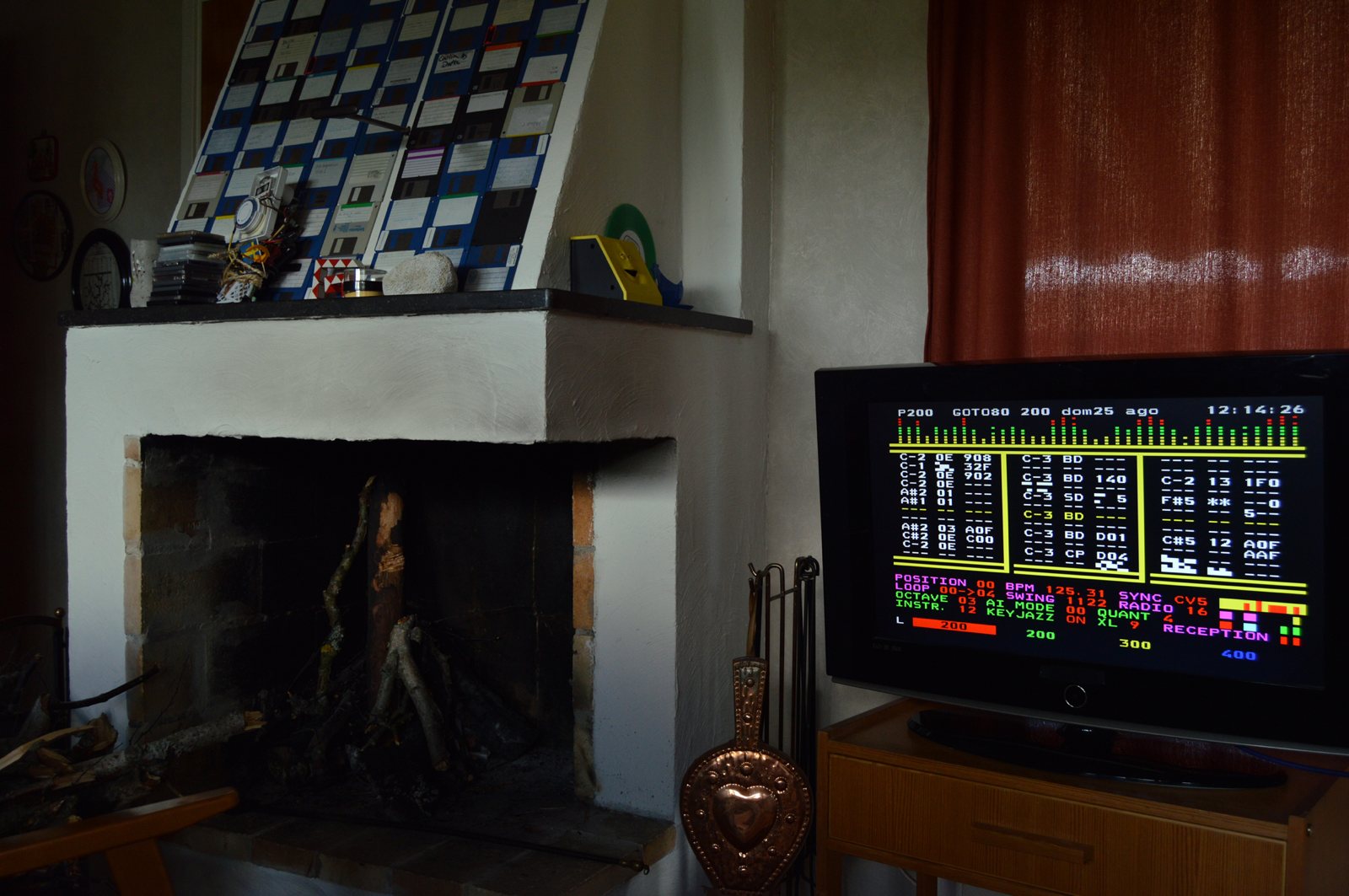This is an image of a photograph taken inside a room with beige walls, giving off a somewhat dark ambiance due to the lack of lighting. In the lower right corner, there's a wooden table with a small drawer, and on this table sits a monitor, which could be a computer screen or a TV. The monitor displays several columns of lines, graphs with yellow numbers, and more code in purple, green, and red fonts, suggesting various settings such as position, octave, AI mode, and quant. Behind the monitor, there's a window adorned with a red curtain. To the left of the monitor, there's a brick fireplace with a white mantle, accompanied by fireplace utensils that appear to be made of copper. The outside of the fireplace is either painted tan or beige, and atop the mantle, there are assorted knickknacks, including candles and a painting leaning against the wall. A poster board with labels contributes to the room’s detailed decor.